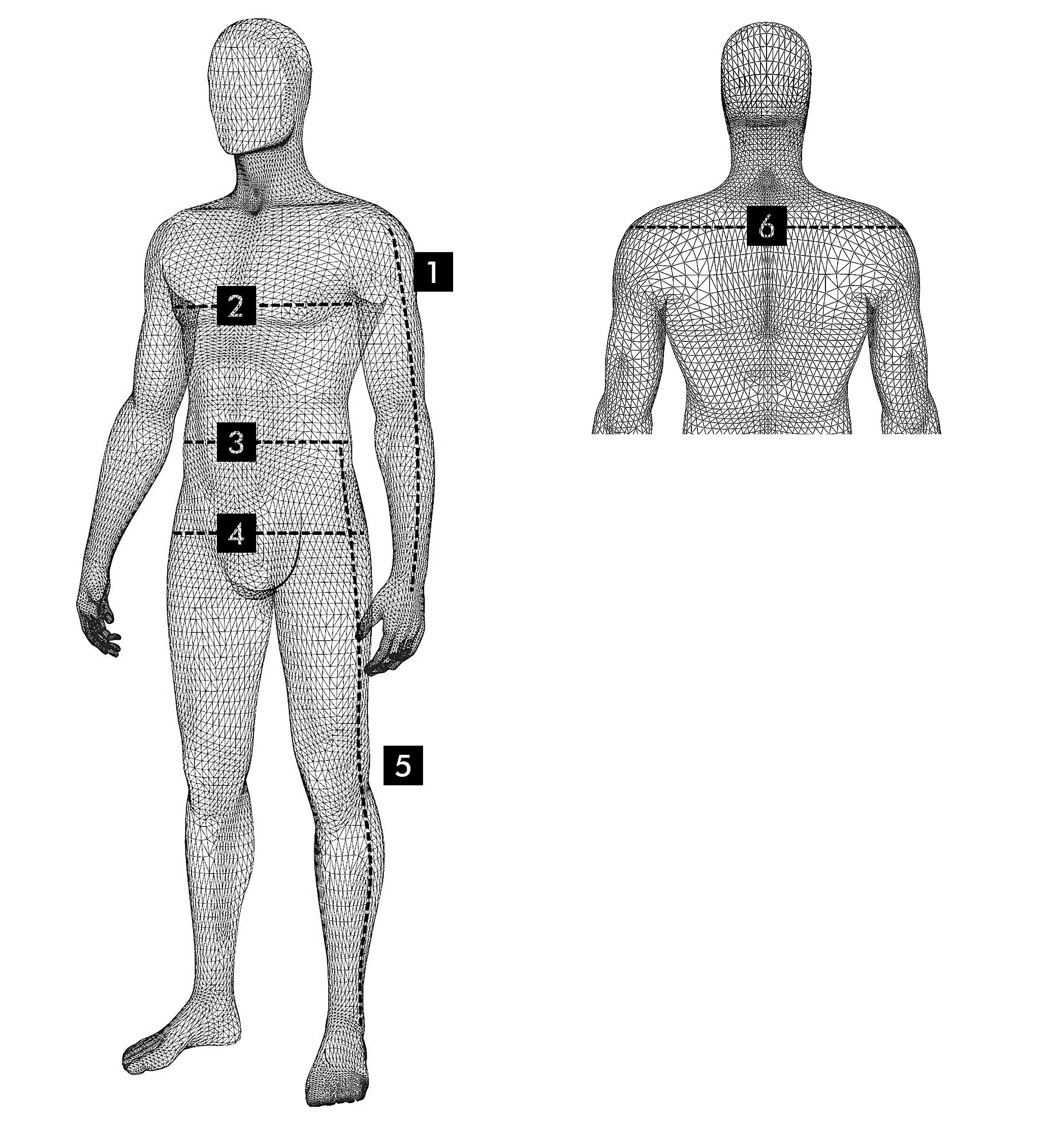This black and white illustration features a detailed diagram of a human figure against a plain white background, presented in portrait orientation. The image is divided into two side-by-side depictions of the body—one full figure on the left and a partial figure on the right.

On the left, the outline of a male human figure stands about five inches high, facing slightly toward the left. It's a basic form without facial features, designed to show measurements of different body parts. Black squares with white numbers inside are used to label these parts, connected by dotted lines. The labels are as follows:
1. The left arm
2. The upper chest
3. The waist
4. The hips
5. The entire length of the left leg.

To the right, a view from the back displays the figure from the head down to just below the elbows. This view cuts off before the legs, focusing on the upper body. One dotted line runs horizontally across the shoulders, marked with the number 6.

This diagram, through its numerical labels and dotted lines, likely serves to indicate specific measurement points, possibly for tailoring or anatomical reference.